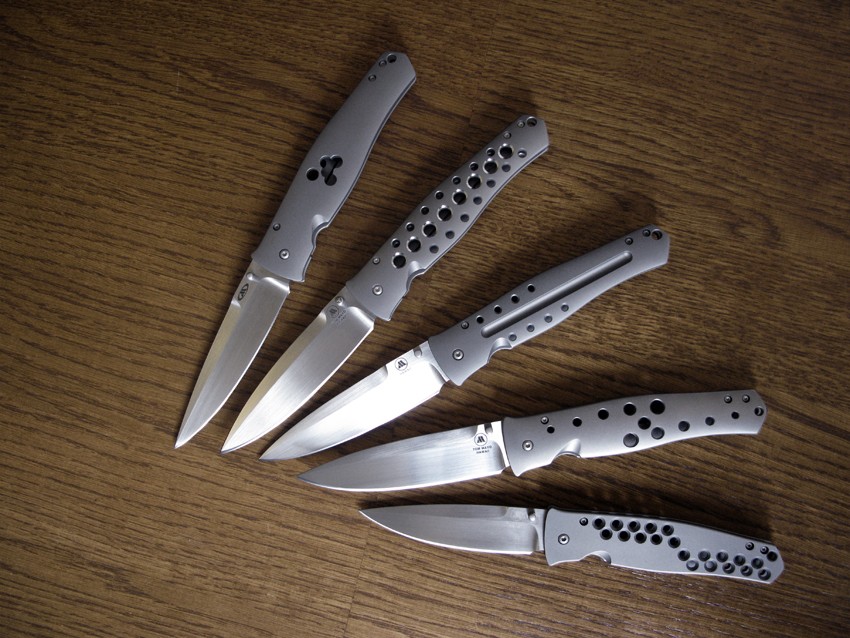This is a detailed overhead color photograph depicting five pocket knives arranged in a fan shape. The knives have sleek, sharp blades made of silver or metal, all pointed towards the lower left corner of the frame. The grey handles of each knife feature a series of regular, circular cutouts, though with varying designs across the knives. The arrangement of the knives is such that their handles spread out towards the upper half of the image, creating a distinctive, fan-like pattern. The knives rest on a dark, brown wooden table with visible grain, adding to the rustic aesthetic. The lighting is mostly dim, but a bright highlight prominently illuminates the center knife, casting reflective glints on its shiny blade.